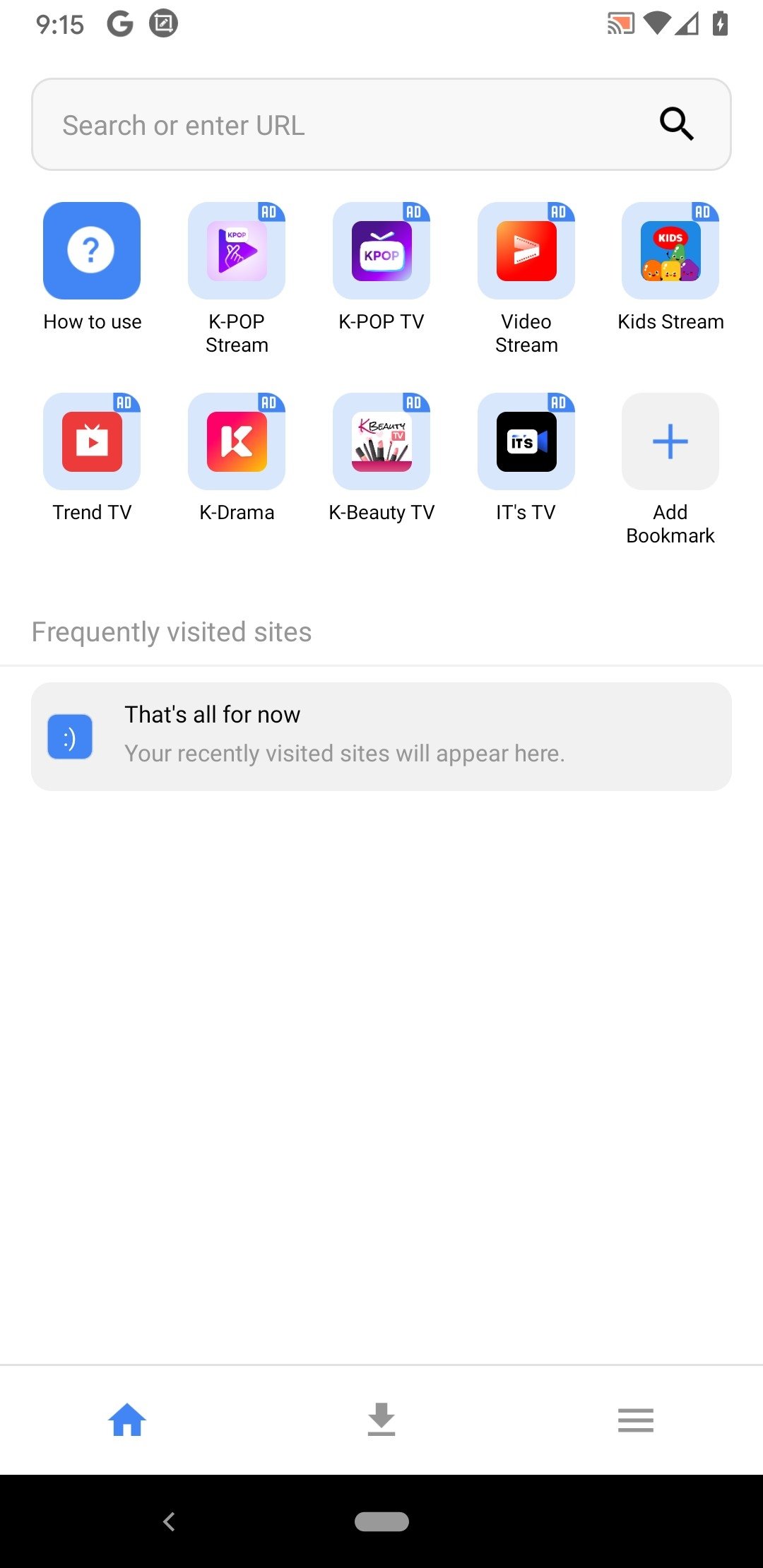This image captures the mobile view of a browser interface on what appears to be an Android device, identified by the typical top-bar icons such as battery level, Wi-Fi signal, and the time reading 9:15. The screenshot showcases a browser window, possibly a Google browser, suggested by the presence of a 'G' logo in the top corner. At the very top is a search bar that reads "search or enter URL".

Below the search bar are two rows containing a total of ten icon "chiclets" that resemble navigation shortcuts:

1. **How to Use**: A blue square with a white circle and a blue question mark in its center.
2. **K-pop Stream**: A blue square with a purple play button, and an “RD” label. 
3. **K-pop TV**: A blue square with an old-fashioned TV icon in purple, also labeled “RD”.
4. **Video Stream**: An orange square with a film reel icon against the blue background.
5. **Kids Stream**: A blue square with three vegetables in orange, yellow, and purple colors.

The second row includes:

6. **Trend TV**: A blue square with an old-fashioned TV icon, featuring a red square and play button.
7. **K-drama**: A blue square with a red ombre icon displaying the letter “K”.
8. **K-beauty TV**: A blue square featuring makeup brushes and the “K-beauty” text within a white square.
9. **It's TV**: A blue square with the word “It's” on top of a camera image set against a black background.
10. **Ad Bookmark**: A gray square with a blue plus sign.

Below these chiclets, a section is marked "Frequently Visited Sites," indicating that recently visited sites will appear in this area, currently accompanied by a blue box with a white smiley face and the text "that's all for now."

At the bottom of the screen, there are three icons: a home icon, a download icon, and a menu icon (depicted as three lines). Additional phone-related icons are found further down the interface, completing the mobile browser view.